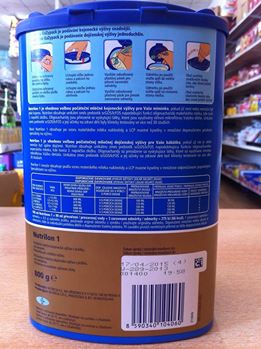In the image, there is a vertical rectangle capturing a close-up of the back of a packaging container. The scene appears to be set in a store, as evidenced by visible aisles, shelves stocked with various products, and a typical retail setting with white, grid-patterned ceilings. At the center of the image sits a blue cylindrical container positioned on a brown countertop. The bottom portion of the container is brown, transitioning to blue at the top. Detailed instructions for product use are displayed prominently on the container's back, along with a barcode situated at the bottom, ready for scanning. The background elements are slightly blurred, keeping the focus on the packaging.